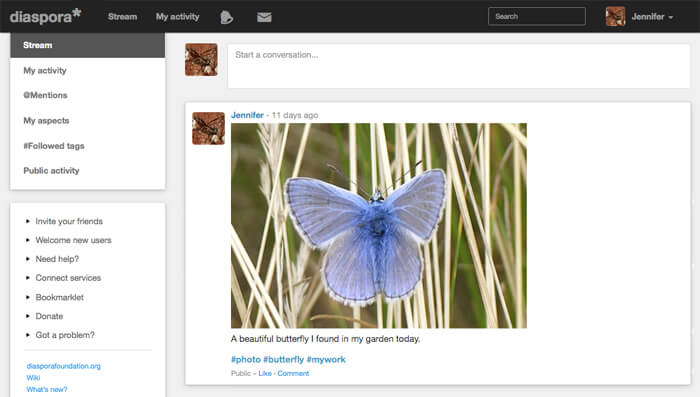Certainly! Here's a detailed and cleaned-up caption for the described image:

---

This image showcases the user interface of Diaspora, a social media or blogging platform. The background mainly features a white color scheme. At the top, there is a long, rectangular black bar displaying the logo "Diaspora" accompanied by a star symbol. To the right of the logo, the menu options include: Stream, My Activity, a bell icon for notifications, an email/message notification icon, a short search bar, and the user name "Jennifer" along with her profile picture of a squirrel.

Below the top bar, on the left side, there is a long vertical menu divided into two sections. The first section contains the following menu items: Stream, My Activity, Mentions, My Aspects, Follow Tags, and Public Activity. The second section lists: Invite Your Friends, Welcome New Users, Need Help, Connect Services, Bookmark, Donate, and Got a Problem. Further down, there is a URL field, followed by a “What’s New” section.

On the right side of the image, occupying a significant portion of the screen, there is a content area divided into two main parts. The top part features a long rectangular box with the prompt "Start a conversation." Below it is a wider rectangular section displaying a user's post. The post is authored by Jennifer, dated 11 days ago. The content showcases a beautiful blue butterfly perched amidst nature, with leaves and stems visible in the background. Jennifer has captioned the photo with, "A beautiful butterfly I saw in my garden today," and included hashtags such as #photo, #butterfly, and #mywork. Users have the option to like or comment on the post.